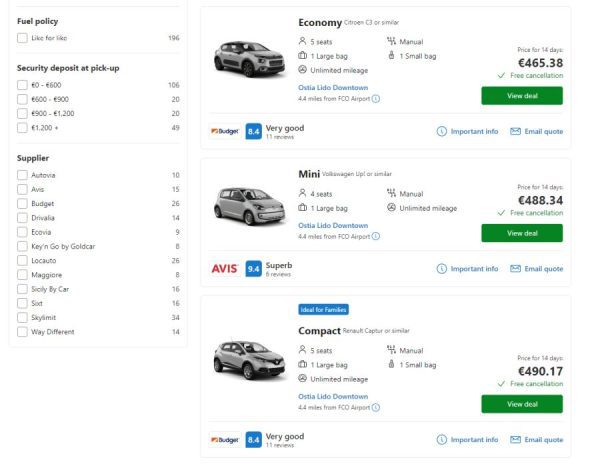A screenshot of a computer screen displaying a comparison of various car rental options based on fuel economy. On the left, there's a column titled "Fuel Policy," with options like "Like for Like" that can be selected, but none are currently checked. Below this, a section labeled "Security Deposit at Pickup" shows a range, likely indicating the number of available cars. The suppliers are listed underneath, featuring rental companies such as Avis, Budget, and Keys Go by Gold Star. 

To the right, the car listings are organized by price and quality. The first car listed is an economy model priced at 468.38 euros, with an option to view more details. A middle entry shows a "Very Good" rated mini from Budget at 488.34 euros, also viewable. At the bottom, a compact car from Avis is available for 490.17 euros, rated as "Superb." Additionally, there's a mention of another very good quality option that is slightly off the current view of the screen.